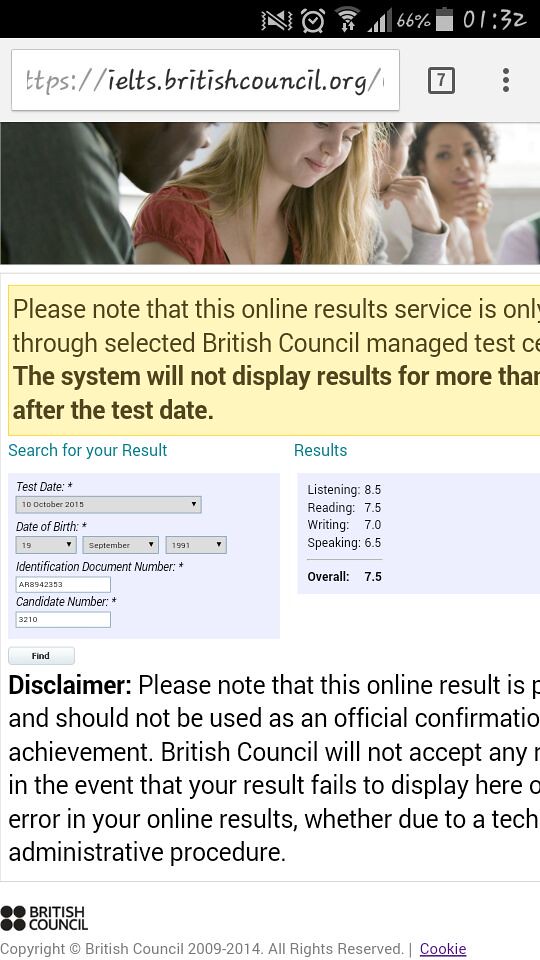The screenshot displays the britishcouncil.org website on a mobile device. At the top of the screen, there is a stock photograph featuring two men and two women engaged in conversation. The text beneath the address bar indicates: "Please note that this online results service is only available through selected British Council Managed Tests..." (with the remainder cut off). There are sections for search parameters where users can input test date, date of birth, identification document number, and candidate number to look up test results. 

Furthermore, the disclaimer details: "Please note that this online result is not to be used as an official confirmation of achievement. The British Council will not accept any claims in the event that your result fails to display here due to technical or administrative errors." The system will only display results for a certain period after the test date. Users can look up results for listening, reading, writing, and speaking sections of their tests.